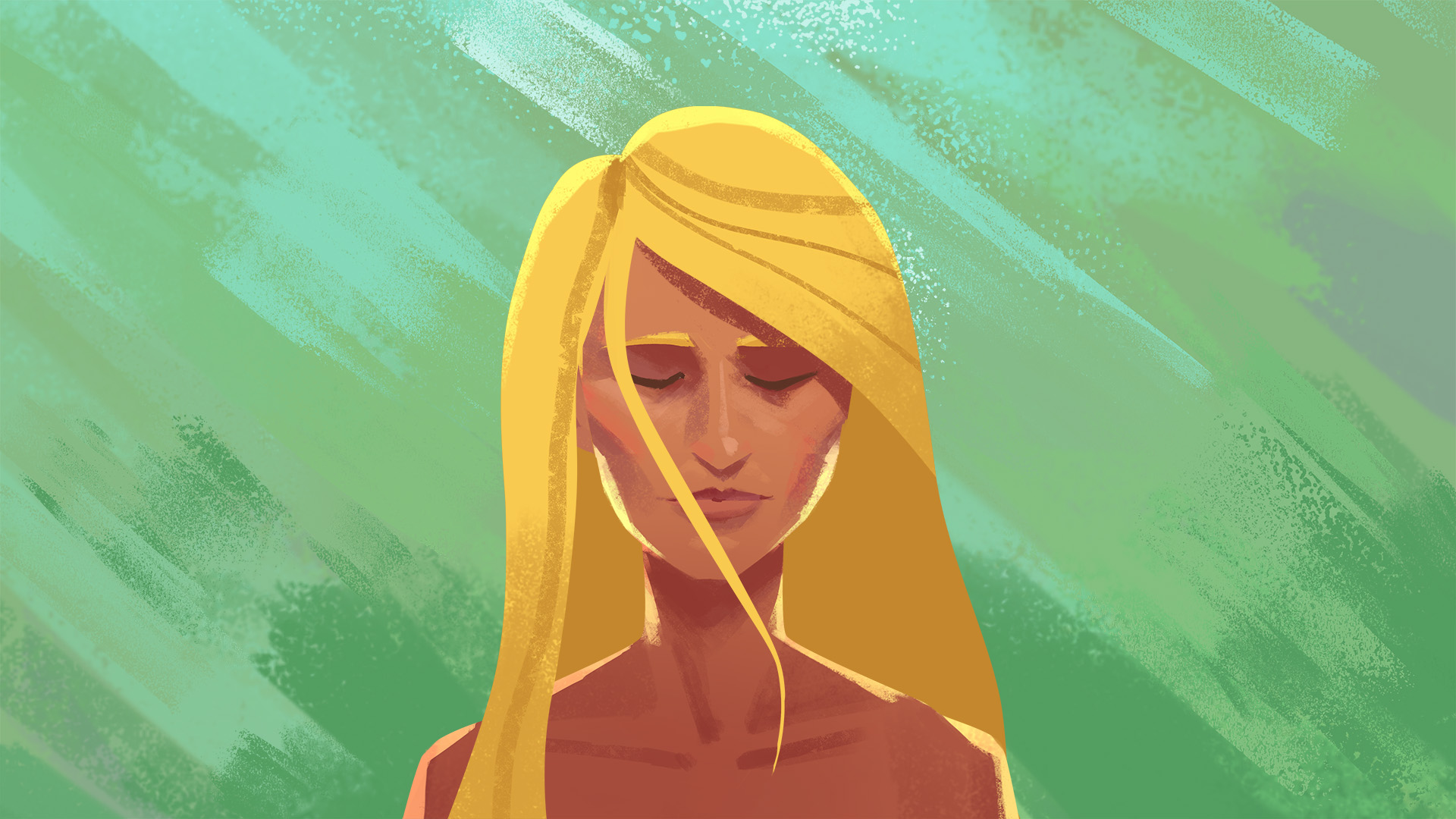This image is a cartoon-style illustration, characterized by a block paint style, depicting a thin, olive-toned tanned woman with a serene expression as she stands in a slanting rain shower. Her bright yellow hair, parted to either side, cascades down her back with a single wavy strand blowing across her face, partially covering one eye and her mouth. The woman has her eyes clamped shut, emphasizing her peaceful, introspective demeanor. Her natural rose-colored lips and shadowed cheekbones, eyes, neck, and collarbones contribute to the subtle shading details. The predominant green background is rendered with thick, multi-shade brushstrokes, slanting diagonally from the upper left to the lower right, with seafoam, light, and dark green hues evoking the imagery of falling rain. The painting's simple yet evocative style leaves the woman appearing possibly naked, with only her head and bust visible, adding an element of vulnerability to the captivating scene.